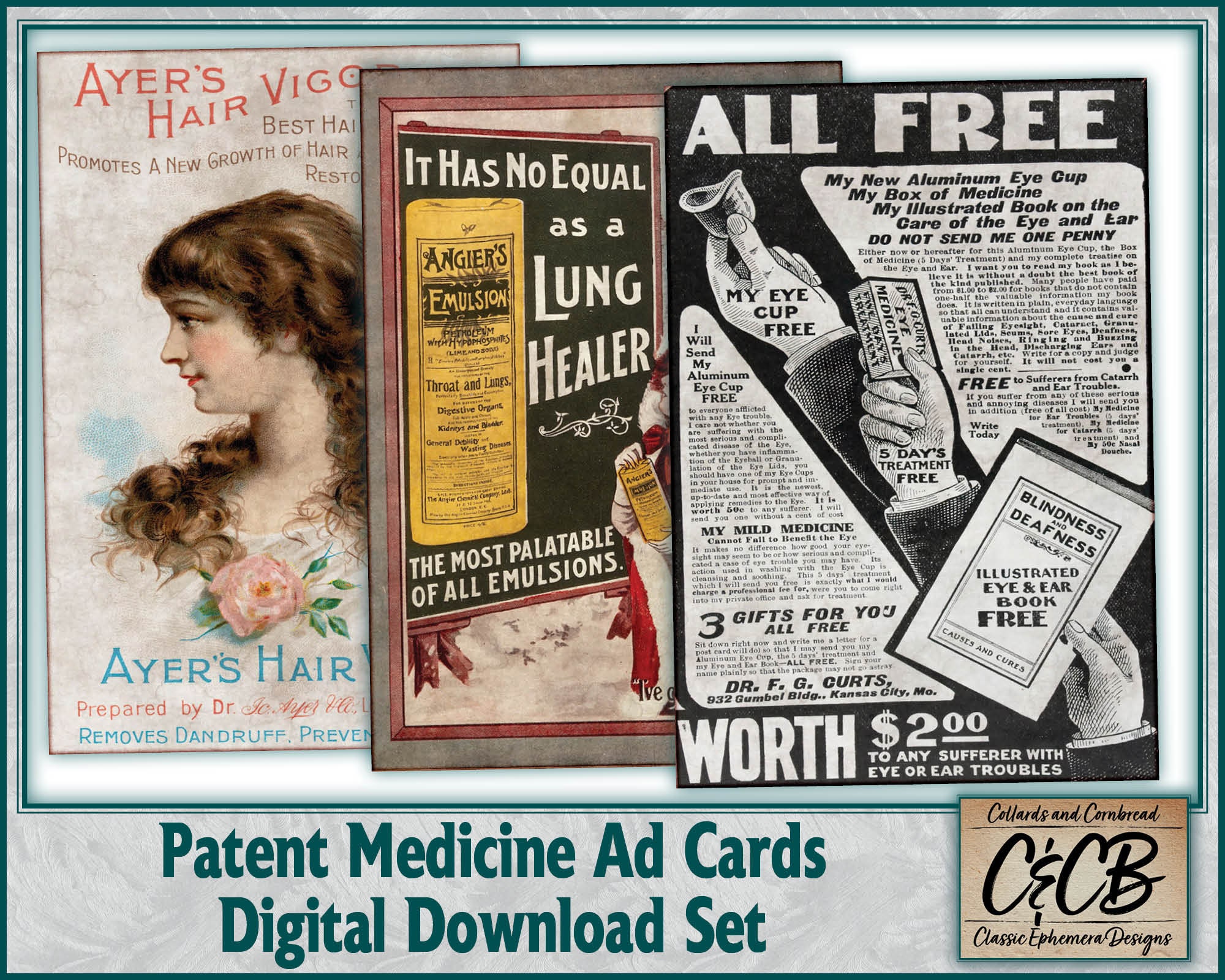The color photo showcases a vintage collection of medical advertisements titled "Patent Medicine Ad Cards Digital Download Set." The composition features three overlapping posters bordered by shades of dark blue. The top-left poster, in color, promotes "Ayer's Hair Vigor," depicting a woman looking left with text claiming the product removes dandruff. The center poster highlights a lung remedy, stating "It has no equal as a lung healer, the most palatable of all emulsions." The right-most advertisement, in black and white, offers a free booklet worth $2 for those suffering from eye or ear troubles. Additional text on the image mentions "Collards and Cornbread, C&CB Classic Ephemera Designs," further emphasizing the vintage aesthetic. The vivid hues include shades of black, blue, brown, light pink, yellow, and white.